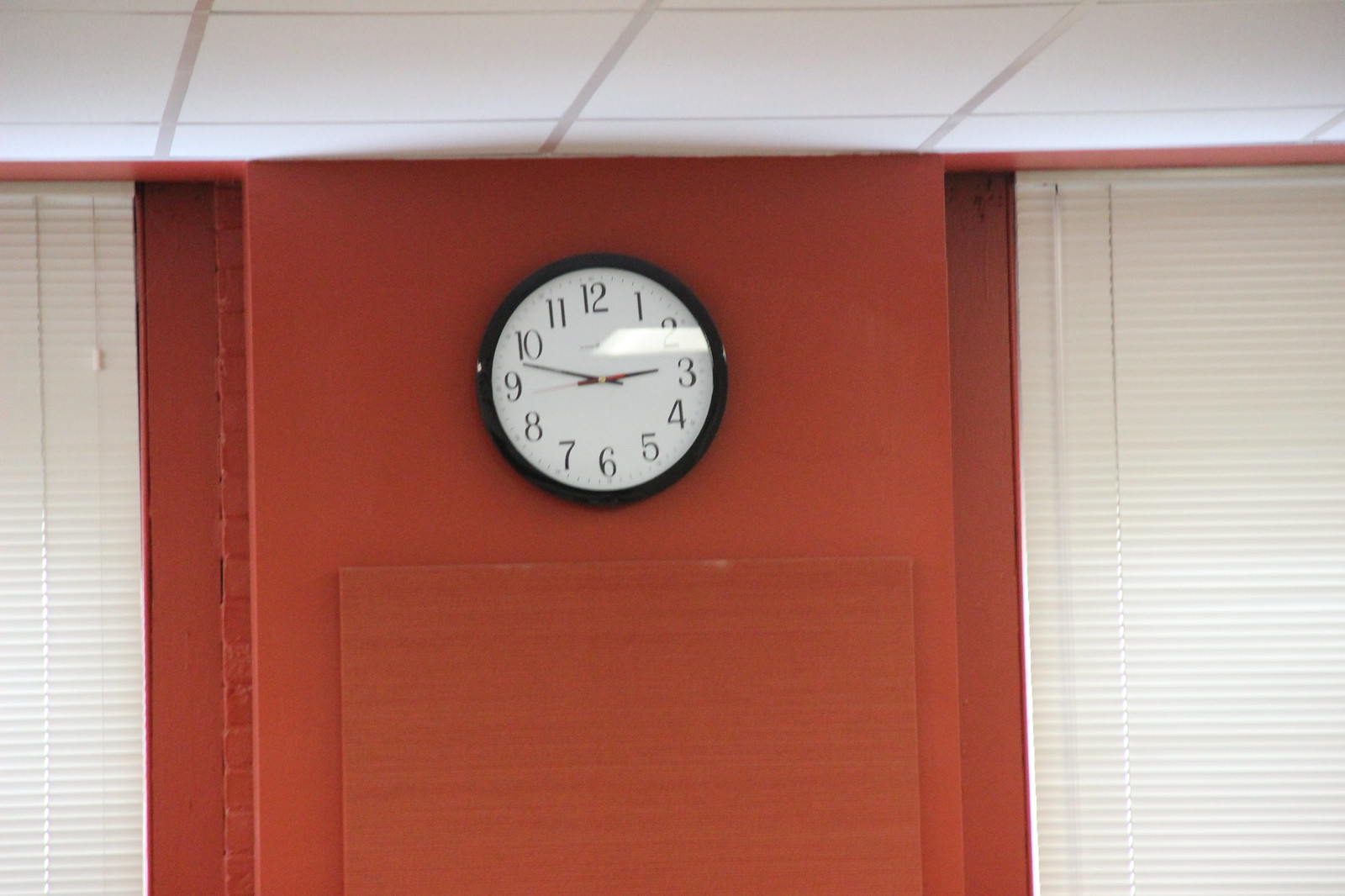In an interior space, a round wall clock is prominently mounted on a red-painted section of the wall. The clock, which displays the time as 2:48, features a black rim, a white face, black numerals, black minute and hour hands, and a red second hand. Flanking the clock are two windows, each covered in white blinds, creating a balanced visual symmetry. Above, part of a white tile drop ceiling is visible, adding to the structured aesthetic of the room. Below the clock, a square panel hints at a covered opening, possibly from an old fireplace. On the far left and right edges of the wall section, rows of bricks are visible, providing a rustic contrast to the otherwise modern interior elements.